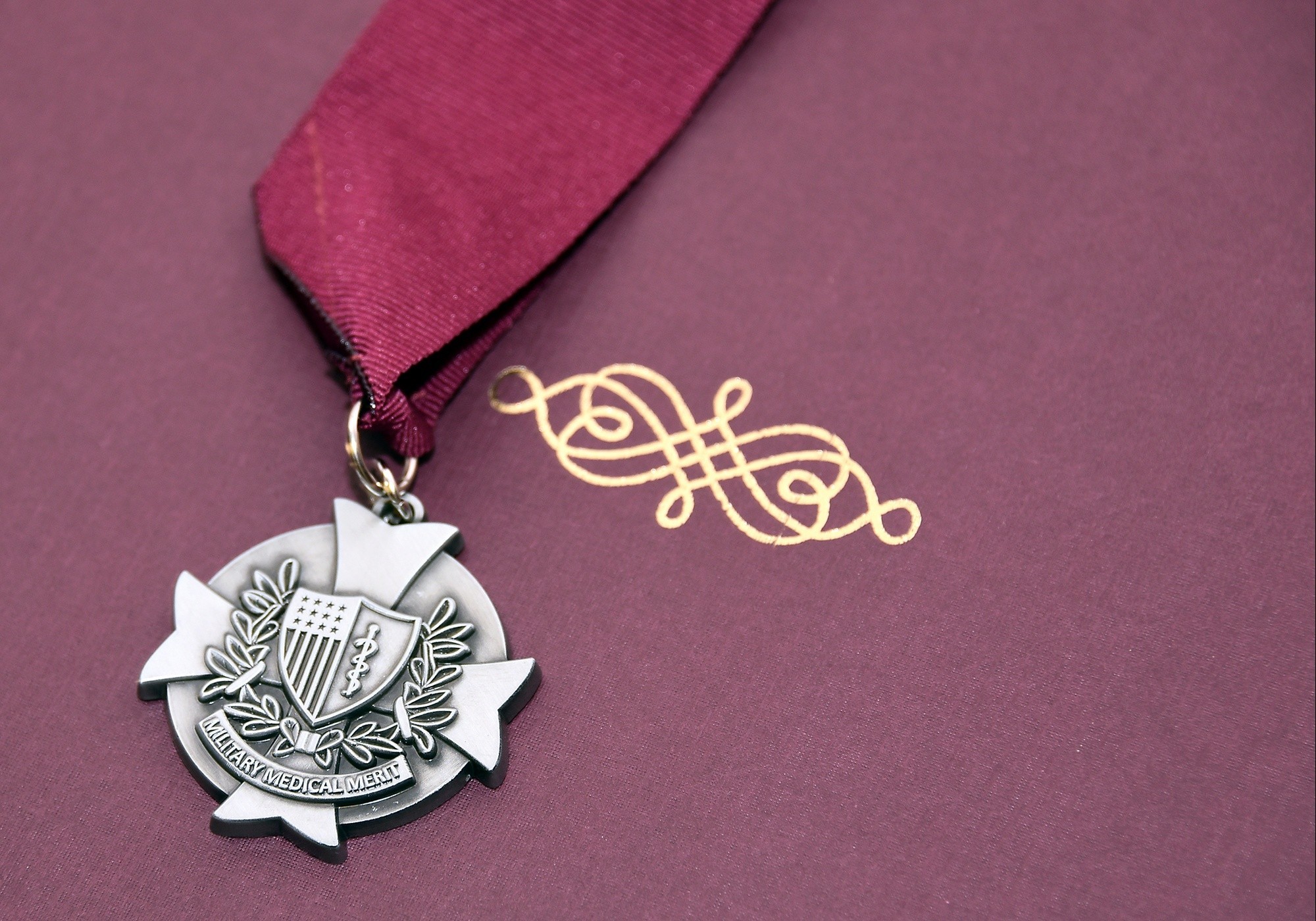In the photograph, a military medal prominently hangs from an amber-colored strap on the left side. The medal is attached to the strap with a gold ring. The silver-colored medal is circular, featuring intricate designs. At its center, the medal displays an image of a shield adorned with stars and stripes on the left side, and a pole with a snake coiled around it on the right side, symbolizing the medical profession. Below this, floral designs add decorative detail. The lower part of the medal features an inscription that reads "Military Medical Merit" in a half-circle. 

To the right of the medal, centered in the photograph, there is an elegant gold-colored etching composed of swirling lines that terminate in circles, with a couple of X's interspersed in the middle. The amber-colored background of the image complements the gold etching, which nearly touches the purple strap from which the medal hangs, creating a striking visual contrast.